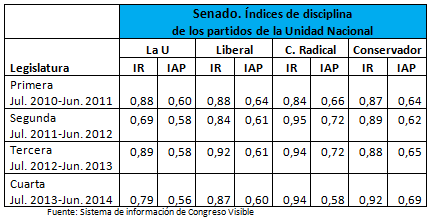The image depicts a detailed chart titled "Senado Indices de Disciplina de los Partidos de la Unidad Nacional," presented in Spanish. This chart is formatted on a postcard-sized card, with a distinctive blue header filled with white text. Below this header, the chart is organized into four primary columns labeled "la U," "liberal," "si.radical," and "conservador." Each of these columns has two sub-columns branching downwards. On the left side of the chart, there’s a vertical heading "Legislatura," followed by four rows representing different legislative periods: "Primera" (Julio 2010 a Junio 2011), "Segunda" (Julio 2011 a Junio 2012), "Tercera" (Julio 2012 a Junio 2013), and "Cuarta" (Julio 2013 a Junio 2014). The chart primarily uses black and white for its text and sections, apart from the blue header. At the bottom, there's a footer that reads "Fuente Sistema de Informacion de Congreso Visible." This card appears to be used for tracking some numerical data related to the mentioned legislative periods and political party disciplines.